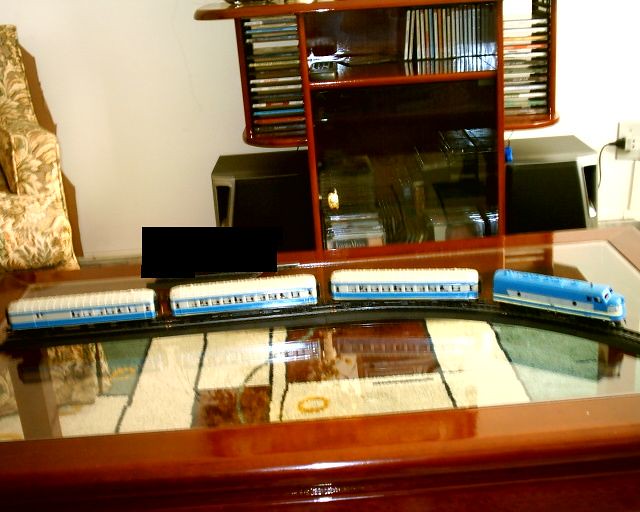In this home setting photograph, a meticulously clean glass-topped desk with a shiny brown hardwood frame serves as the focal point. Situated on the desk is an intricate black toy train track hosting a blue locomotive followed by three white cabooses adorned with blue stripes and windows. The desk is complemented by a decorative rug featuring a pattern of white, brown, and green squares. Behind the desk, a white wall offers contrast to a packed entertainment center filled with videos, DVDs, and CDs, and flanked by two large black speakers. A decorative chair with a light green and yellow embroidered leaf design sits to the left, adding an extra touch of warmth to this homely scene.